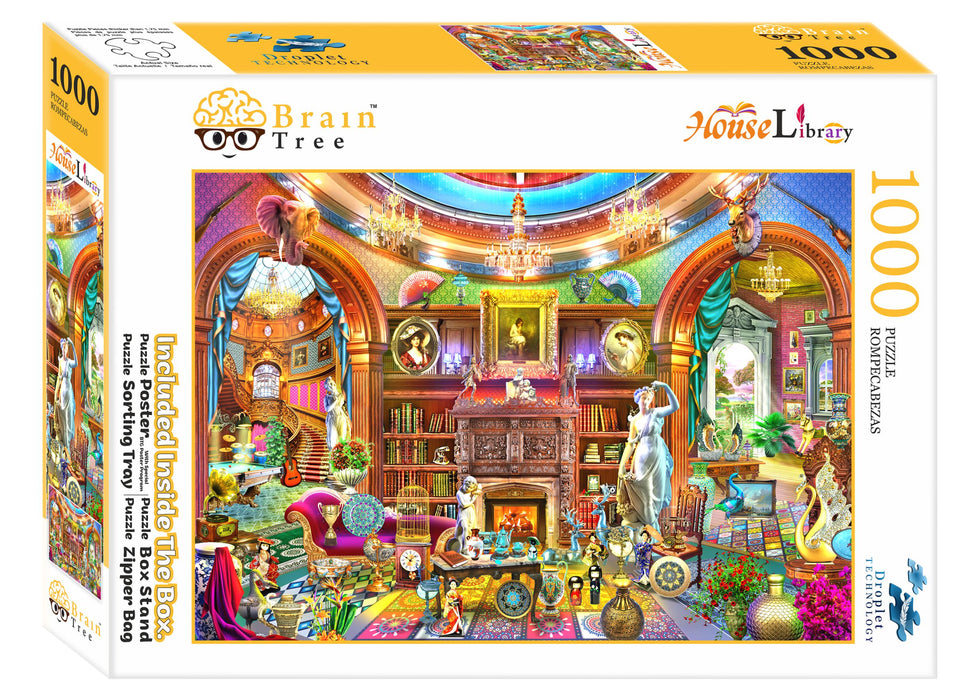The image showcases the front and sides of a 1,000-piece puzzle box by Braintree, distinguished by its yellow brain logo with glasses and a smile. The box is set against a plain white background. Prominently featured is a vibrant illustration depicting an intricate, opulent room resembling a library or stately mansion. The room's decor is lavish, filled with statues, chandeliers, and an array of colorful, ornate objects ranging from vases and books to trophies and clocks. There are flowering plants, patterned rugs, and a gold staircase with a guitar at the base. Arched entryways lead to side rooms brimming with extravagant items. Text on the box highlights the inclusions: a puzzle poster, a box stand, a sorting tray, and a zipper bag. The myriad of colors—reds, greens, golds, teals, purples, and more—set a maximalist, antique ambiance, making the puzzle both visually stimulating and challenging.